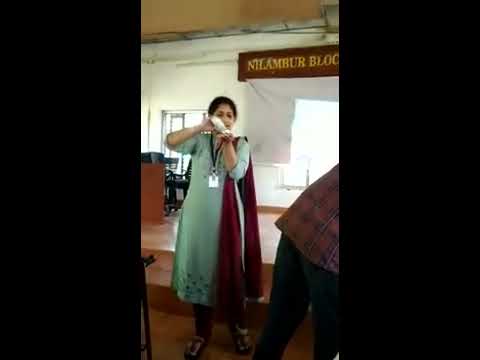The photograph captures a woman of Middle Eastern or South Asian descent standing indoors, seemingly in front of a stage under a sign that reads "Nilambur BLOCK." She is dressed in a traditional green salwar kameez with a long, light teal dress that has three-quarter sleeves and is trimmed with darker green spots at the bottom. She complements her outfit with brownish pants and sandals featuring leather straps. Draped over her right shoulder is a long burgundy scarf that adds a splash of color to her ensemble. Around her neck hangs a dark lanyard with a white tag, possibly a business card. The woman is holding a white tube in her right hand and appears to be pouring its contents, potentially lotion, into her left hand. To her right, partially out of frame, is another person bending over, wearing a dark maroon shirt with vertical dark markings and black pants. The backdrop features red-tiled flooring and white walls, adding to the indoor ambiance of the setting.